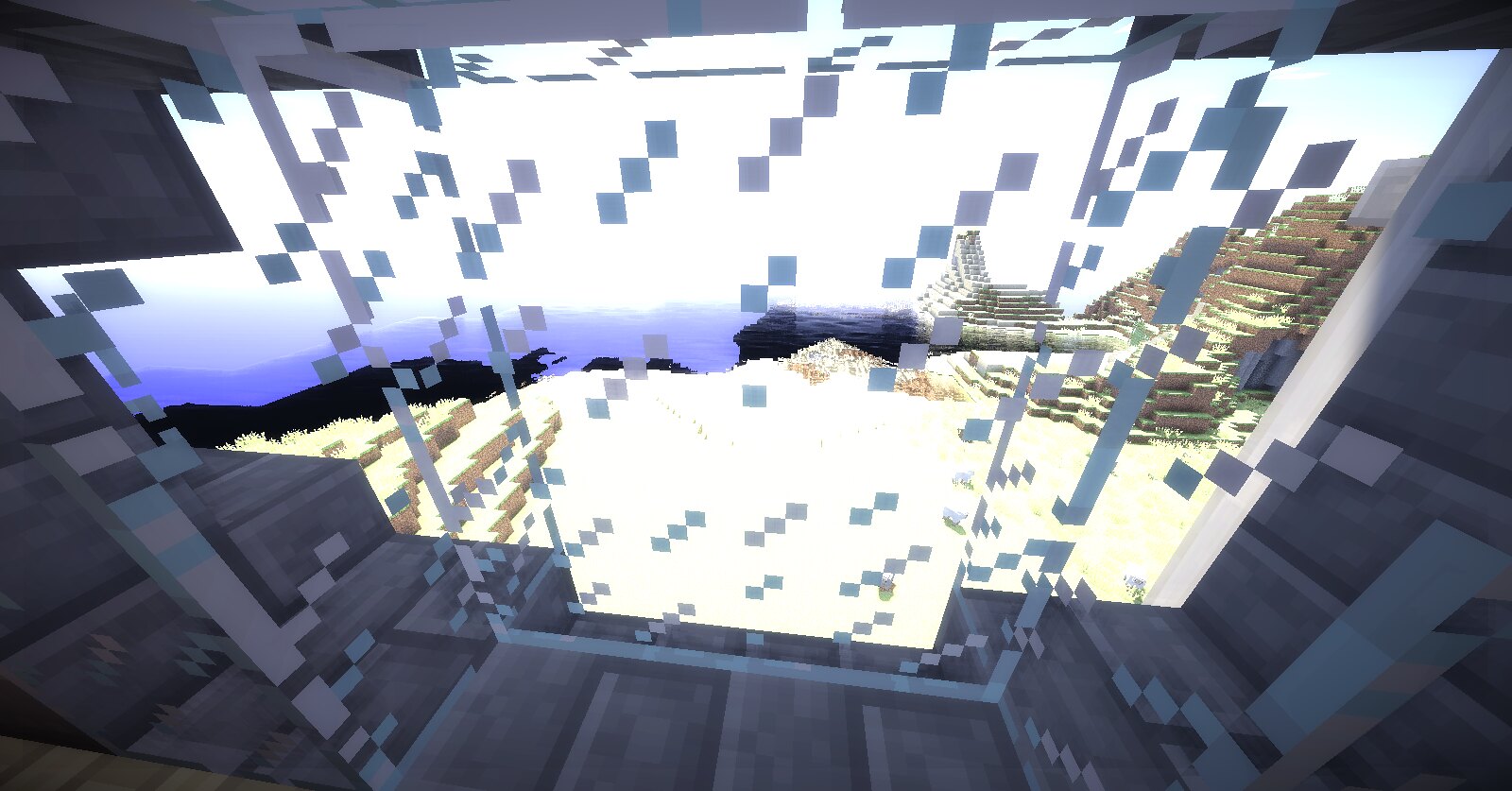This screenshot from the video game Minecraft showcases the distinctive blocky graphics typical of the game. The image captures a scenic view from inside a structure, looking out through a transparent glass block window. The windowpane, identifiable by its translucent quality and strategically placed blue and gray squares simulating light reflections, offers a glimpse of the outside world. The landscape features a gently sloping hill constructed from brown blocks topped with a thin layer of green, portraying grass. Bright, sunlit ground stretches across the exterior, contrasting with patches of blue water that has hints of black coloration, likely indicating depth or shadow in the water. The immediate vicinity outside the window is marked with varying shades of gray, perhaps denoting stone or cobblestone, adding to the game's iconic pixelated aesthetic.